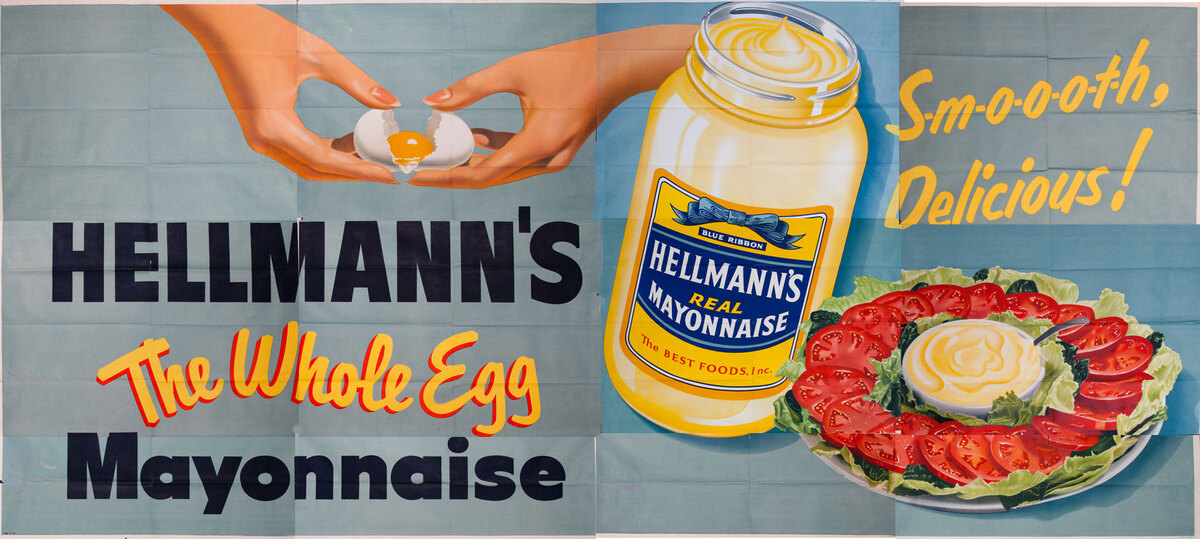This image depicts a vintage-style advertisement for Hellmann's Real Mayonnaise, reminiscent of the early 1940s. The backdrop features a grid of slightly varied bluish-gray and light blue hues, resembling unfolded tissue paper. Central to the ad, two hands are shown cracking an egg. Beneath this, in large, black, capital letters, the word "Hellmann's" is displayed prominently. Below it, in yellow, cursive letters with a solid red drop shadow, is the phrase "the whole egg," followed by the word "mayonnaise" in large black print.

On the left side of the image, there is a distinctive jar of Hellmann's Real Mayonnaise with a yellow label and white text adorned by a blue ribbon. To the right of the mayonnaise jar, there is a round serving plate arranged with lettuce and sliced tomatoes circling a small bowl or ramekin that contains a spoon dipped in creamy mayonnaise. Above this salad plate, in yellow text with a handwritten style, are the words "Smooth - Delicious," with "Smooth" having a dash between each letter. This meticulously detailed composition captures the essence of a bygone era's advertisement aesthetic while emphasizing the key elements of the Hellmann's brand and its wholesome ingredients.